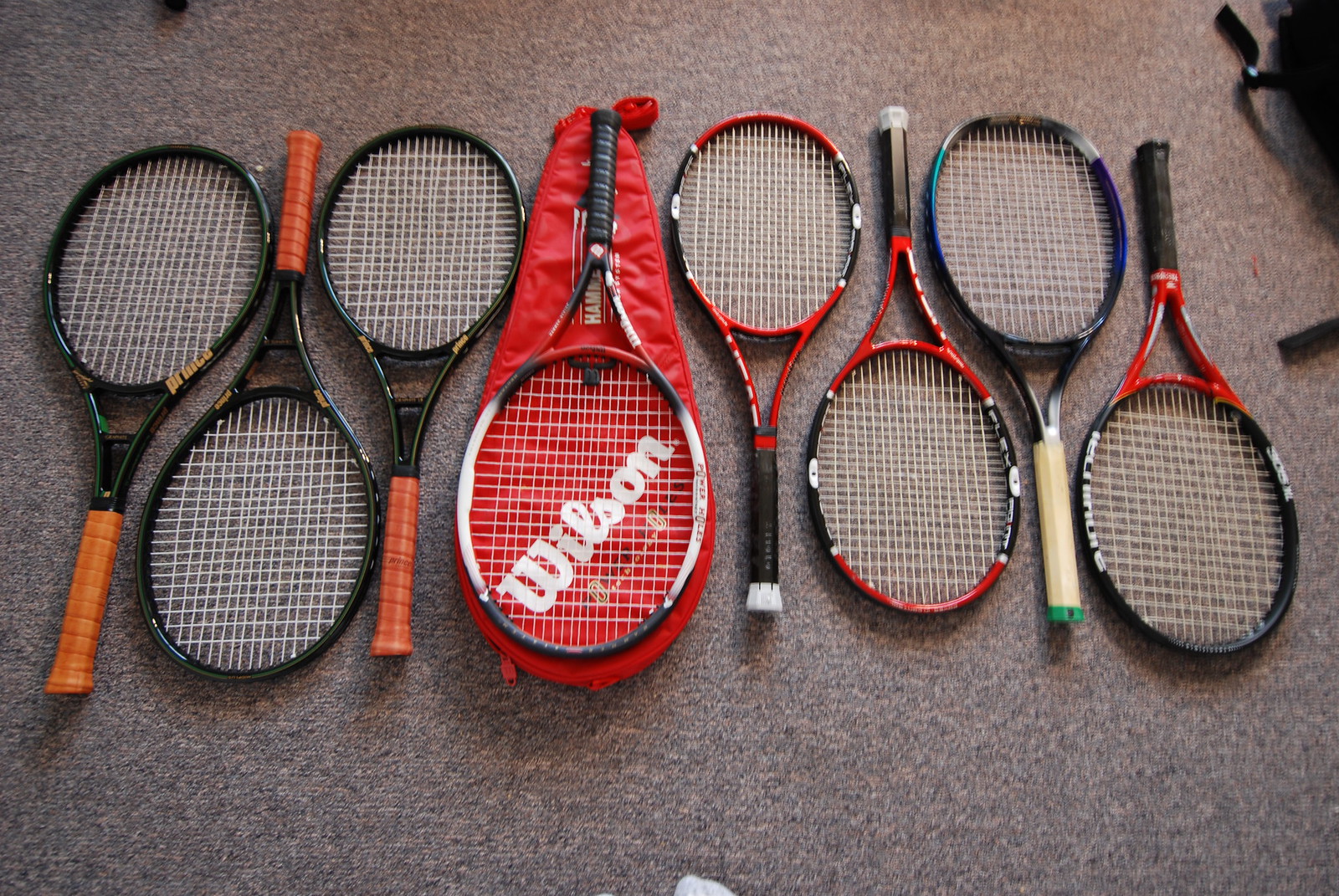The image features eight tennis rackets arranged neatly on a grayish-brown carpet. They are laid in an alternating pattern, with the first racket facing up, the second facing down, and so forth. Among the rackets, the fourth one from the left stands out as it rests on a red Wilson cover with the Wilson logo scripted in white cursive lettering. While three of the rackets are predominantly black with tan handles, another three are a combination of red and black. One racket is black with blue accents and has a natural-colored handle with a green tip. Additionally, in the upper right corner of the image, there is a partial view of what appears to be a black bag or rucksack, along with a bit of white visible in the lower corner. The detailed arrangement and colors of the rackets create a visually appealing and organized display.